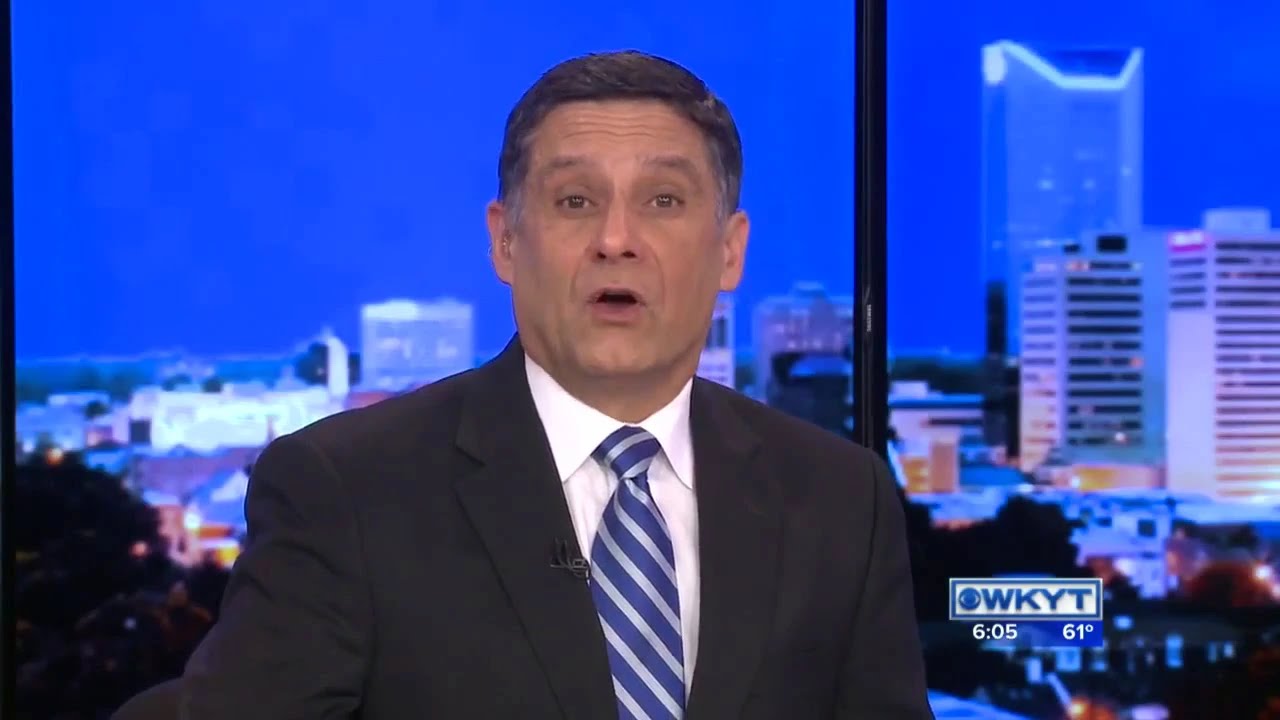This image appears to be a still from a local news broadcast featuring a news anchor positioned centrally on the screen. The man, likely in his 50s or 60s, has short, dark hair with visible gray streaks, particularly on the sides. He has a clean-shaven face with a slightly open mouth, captured mid-sentence, giving him a surprised or action-oriented appearance. He is dressed in a black business suit, complemented by a white collared shirt and a blue tie adorned with gray stripes. A microphone is clipped to his sports jacket, indicating he's actively reporting. Behind him, the background showcases a cityscape, including skyscrapers, office buildings, trees, and cars. In the lower right-hand corner, the channel logo "CBS" and the station identifier "WKYT" are visible in blue font. Below this, white text displays the time, "6:05," and the temperature, "61 degrees."